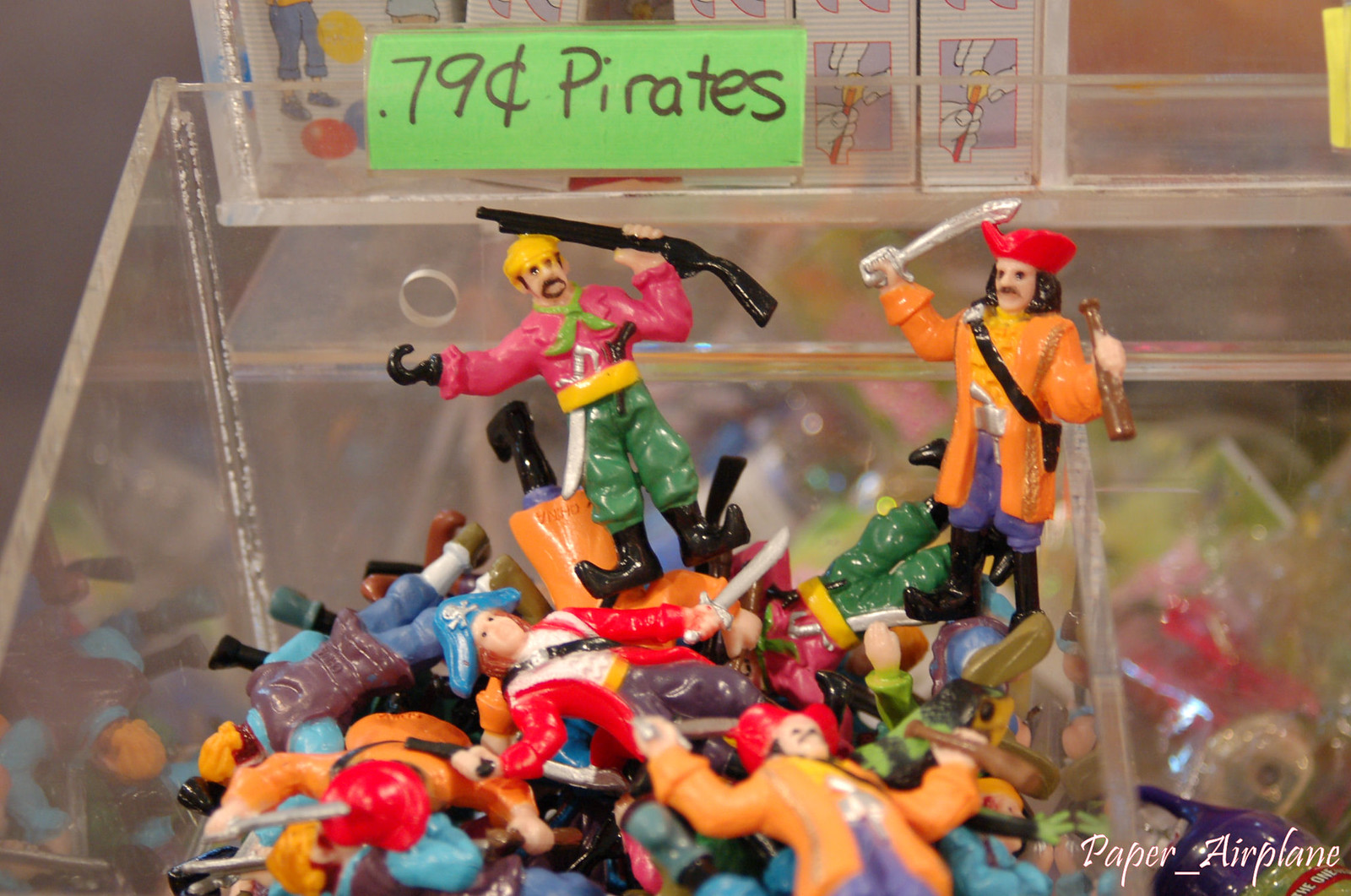The photograph is a rectangular, somewhat aged image, taken indoors in what appears to be a store or a flea market. It features a clear plastic bin filled with various colorful pirate figurines, seemingly made of rubber. Inside the bin, a myriad of colors such as orange, red, blue, green, and black catch the eye. The green label at the back of the bin is inscribed with "79 cents pirates" in black marker.

Among the assortment of toy pirates, two figures stand out prominently. The first pirate, on the left, wears a pink top, a yellow headband, and a yellow belt, with a sword tucked into it. His green pants are paired with boots, and he brandishes a black long gun while his other hand, a black hook, is visible. The second pirate, positioned to the right, is clad in an orange jacket, red pirate hat, and purple pants. He holds a sword in one hand and a bottle of beer in the other, with a pistol tucked into his silver belt and black boots completing his ensemble.

At the bottom right corner of the photograph, white overlay text reads "paper_airplane," adding a modern touch to the vintage feel of the image.